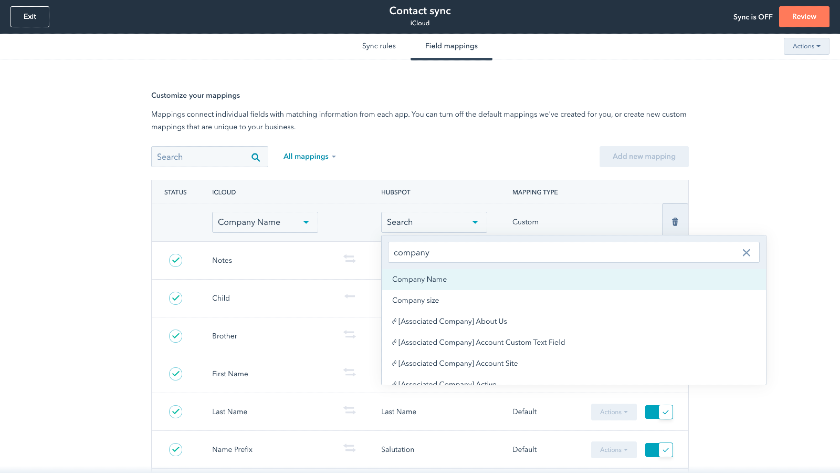A screenshot is displayed with a sleek black banner stretching across the top. The banner prominently features the word "Exit" in white text on the far left, "Contact Sync" in the center, and "Review" on the far right. Notably, "Sync is off" is also indicated on the far right of the banner. 

Just below this banner, text reads "Five-Year Rules and Field Mapping" in a very light and somewhat blurry font. Directly beneath this, more legible text advises, "Customize your mappings. Mappings connect individual fields with matching information from each app. You can turn off the default mappings we've created for you or create new custom mappings that are unique to your business."

Toward the lower left, a search bar is visible next to a drop-down menu labeled "All Mappings.” Below this section, in a light gray tab with black text, the fields are categorized as "Status," "iCloud," "HubSpot," "Mapping Type," "Company Name," "Search," and "Custom." Additional search bars for "Company Name" and "Company Size" are positioned beneath these headings. The overall layout is designed for easy navigation and customization of data mappings.